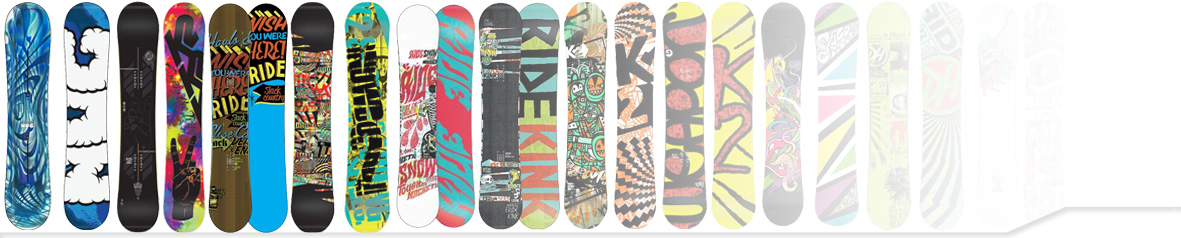The photograph displays a landscape-oriented graphic featuring a diverse collection of approximately 18 to 20 snowboards, each shown upright on their ends and side by side. Each snowboard showcases a unique, artistic design, ranging from blue and green swirls to a design featuring a bug in a cloud shape, along with several brand logos such as K2 and Ride King. The designs are highly varied and eye-catching, with one notably featuring a vibrant tie-dye pattern labeled "K2." As the row extends from left to right, the snowboards gradually fade into a white fog, giving the impression that they vanish into the distance.